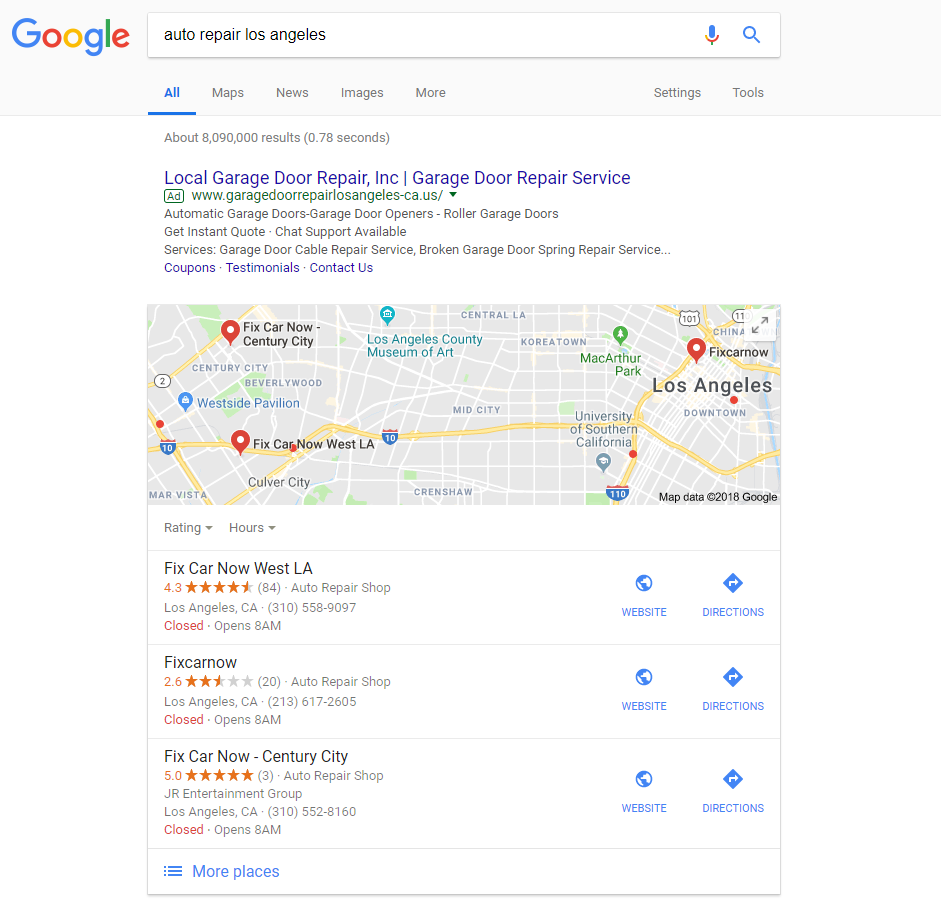A Google search page for "auto repair Los Angeles" is displayed. At the top, a gray rectangular bar features the Google logo on the left, with the iconic blue "G," red "O," orange "O," blue lowercase "g," green lowercase "l," and red lowercase "e." To the right of the logo, a search bar with the query "auto repair Los Angeles" in black text is centered.

Directly below the search bar, a navigation menu highlights "All" in blue and underlined. To the right, unhighlighted gray options include "Maps," "News," "Images," "More," "Settings," and "Tools." 

The main content area has a white background, beginning with search result metrics: "About 8,090,000 results (0.78 seconds)" in gray. The first result is a blue link for "Local Garage Door Repair, Inc. - Garage door repair service" with a URL, "www.garagedoorrepairlosangeles.ca.us," followed by a downward-facing arrow. The description beneath highlights services in gray like "automatic garage doors," "garage door openers," "roller garage doors," and "cable repair service." Links for "coupons," "testimonials," and "contact us" are in blue.

Below, a snippet of a small map marks locations of auto repair shops with three location dots. The first listing, "Fix Car Now - West LA," displays a rating of 4.3 stars in orange, 84 reviews, and provides details like "auto repair shop, Los Angeles, California" and a phone number "310-558-9097" in gray. It indicates "Closed" in red and "Opens 8 AM" in gray, with buttons for "Website" and "Directions" to the right.

Next, "Fix Car Now" is listed with a 2.6-star rating, 20 reviews, address details, and phone number "213-617-2615" in gray, along with similar "Website" and "Directions" buttons.

A third listing for "Fix Car Now - Century City" features a perfect 5-star rating, three reviews, and address and contact information "310-552-8160" in gray, showing "Closed" in red and "Opens 8 AM" adjacent to "Website" and "Directions" buttons.

At the bottom left, three horizontal blue lines appear next to a "More places" link in blue, suggesting additional auto repair locations in Los Angeles.